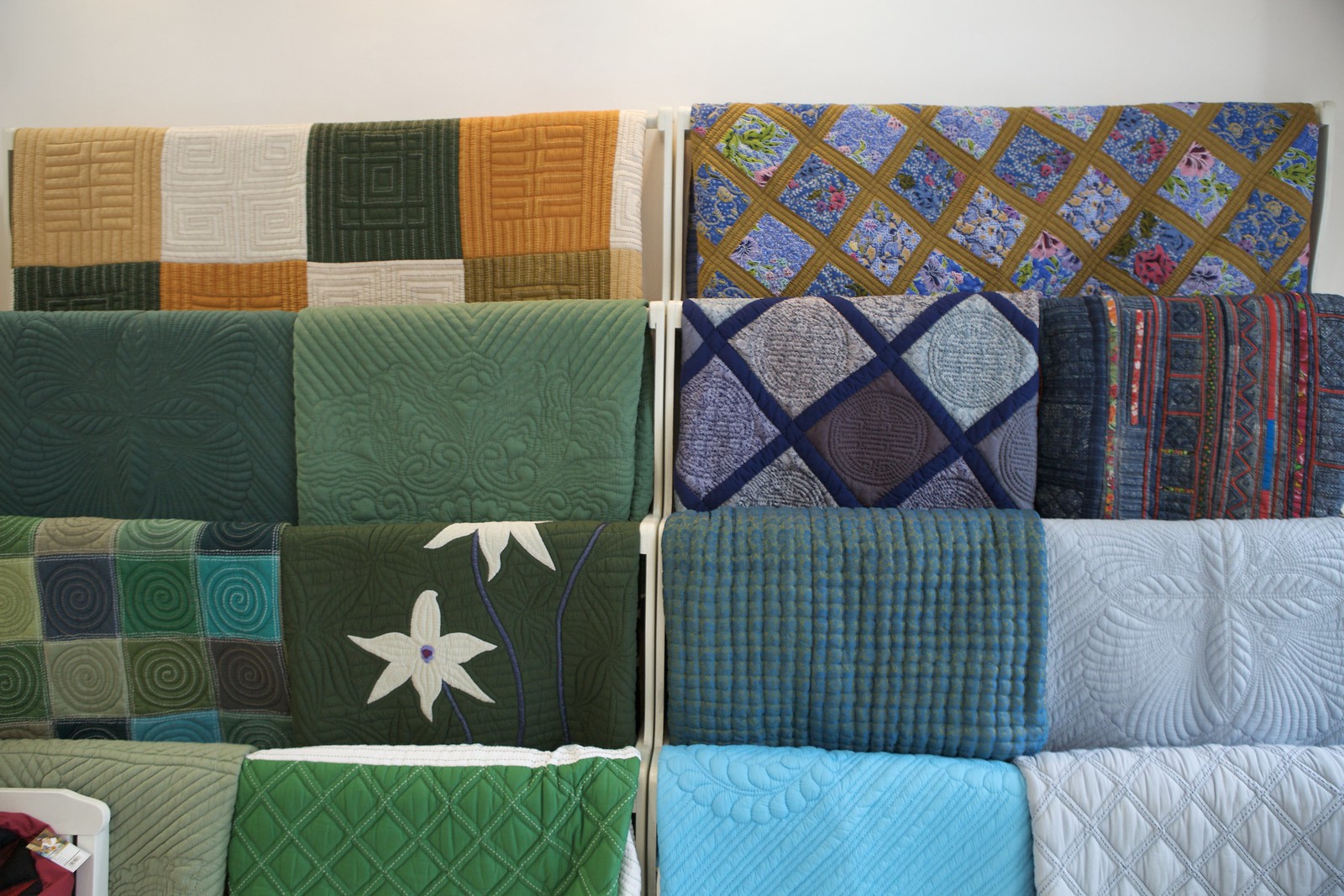This color photograph showcases a detailed display of rugs or throws arranged on shelving units against a white back wall. The display features an overlapping arrangement across horizontal bars with visible white shelving edges, framed by a grey top background.

The top left section displays throws in green, orange, brown, and fawn-colored squares, each with embossed designs. Adjacent, there is a throw with a brown diamond lattice and blue abstract print. Below these are four narrower throws: two green ones with embossed designs (dark green on the far left, then a lighter green), followed by a dark blue throw featuring lighter blue or purplish diamonds with embossed circles, and an abstract-patterned throw on the far right.

The following row exhibits various blue and green squares with embossed circles, beside a dark green throw adorned with white-petal flowers. Proceeding down, there is a blue throw interwoven with a green check, and a grey throw with an embossed petal design. 

At the display's bottom, a pale green throw with a diagonal line design appears next to a green throw and a light blue one with a circular embossed pattern. To the right, a grey throw features dark grey diamonds. The right side's topmost throw is blue with gold stripes creating a box-like center pattern. Underneath, there's a light blue throw with darker blue trim and a white floral-patterned throw. The bottommost rows house a teal blue throw next to a white one, completing the intricate array of patterns and textures.